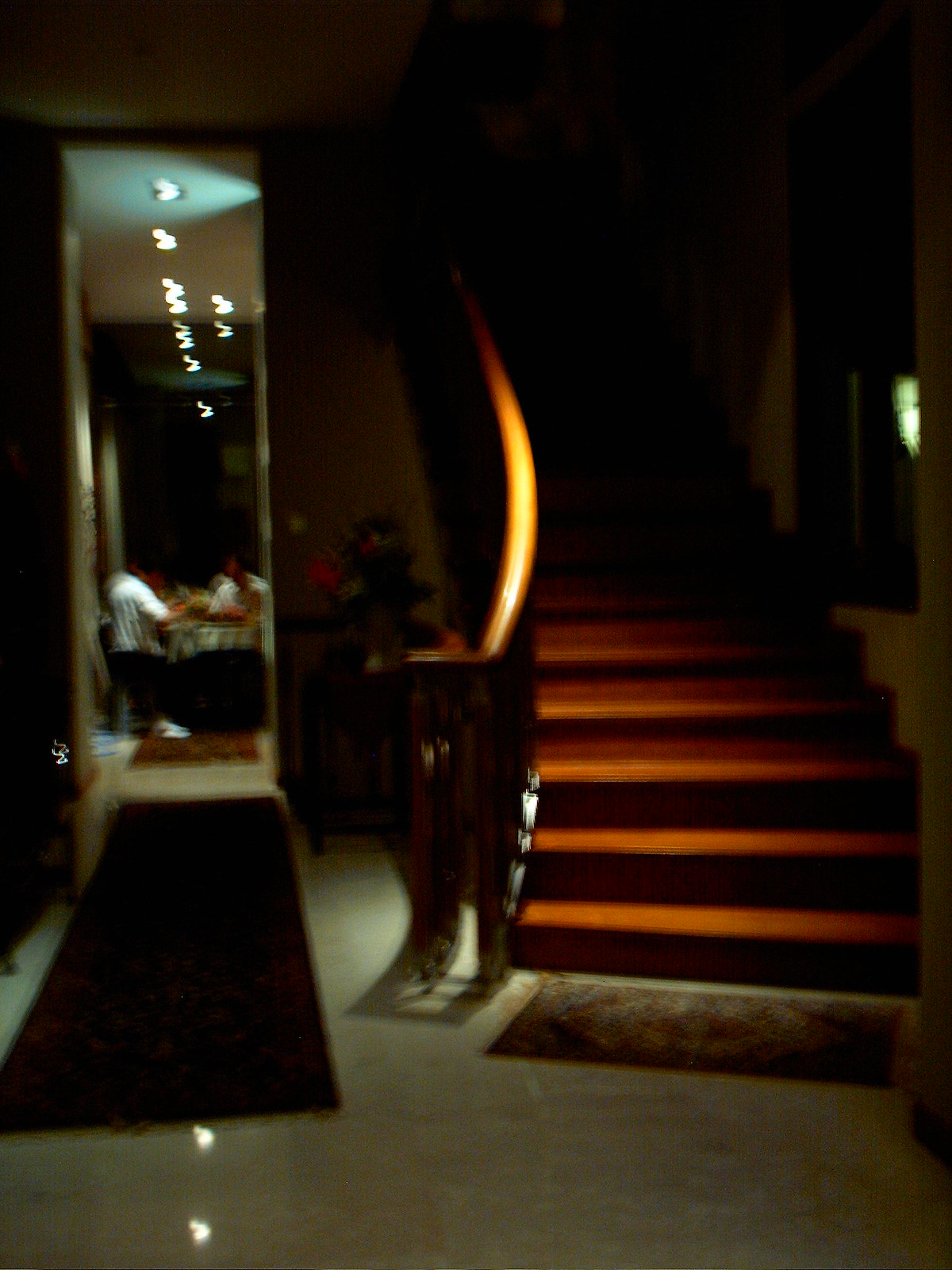The picture shows a dimly lit interior, likely a home's entryway, characterized by glossy marble or shiny tile floors reflecting a bit of available light. On the left-hand side, there's a long carpet runner extending down the hallway. At the bottom of a curved wooden staircase, which ascends into darkness, sits a small rectangular rug. The staircase, edged with a wooden banister, features steps that possibly have reddish wood or are covered in red carpeting. As the staircase ascends, it gets progressively darker until it fades into the shadows. There may be a window on the right-hand wall, providing minimal natural light beside the staircase. In the background, beyond the hallway on the right, a dining area is visible, where a couple of people wearing white T-shirts are seemingly having a meal at a table with a white tablecloth. The image captures some overhead ceiling lights, though the overall illumination is quite faint, adding to the photo's blurred and shadowy appearance.